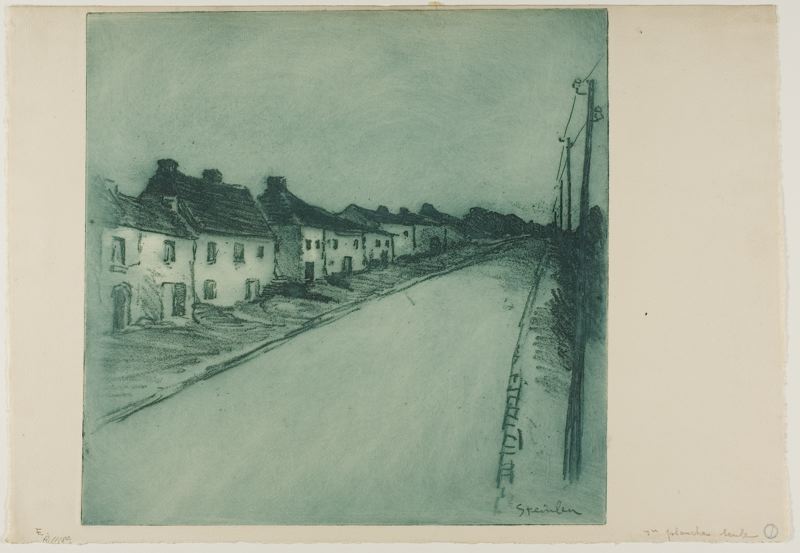This artwork is a detailed pencil or charcoal drawing primarily in black and white, with a subtle greenish or bluish tinge to the shading. The composition is enclosed within a square frame and a faded matte border. The image features a row of two-story houses with black roofs, aligned along the left side of a lightly shaded road and pavement. Notably, each house has chimneys, windows, and doors, depicted with a moderate level of detail. On the right side of the road, there's a telephone pole with power lines extending across the sky, which is lightly shaded with clouds. The artist has employed an interesting perspective technique, causing the buildings to diminish in size as they recede into the distance. The drawing includes the artist's signature, although difficult to read, located at both the lower left and lower right corners, with some suggestion that the name "Tin Ben" appears.